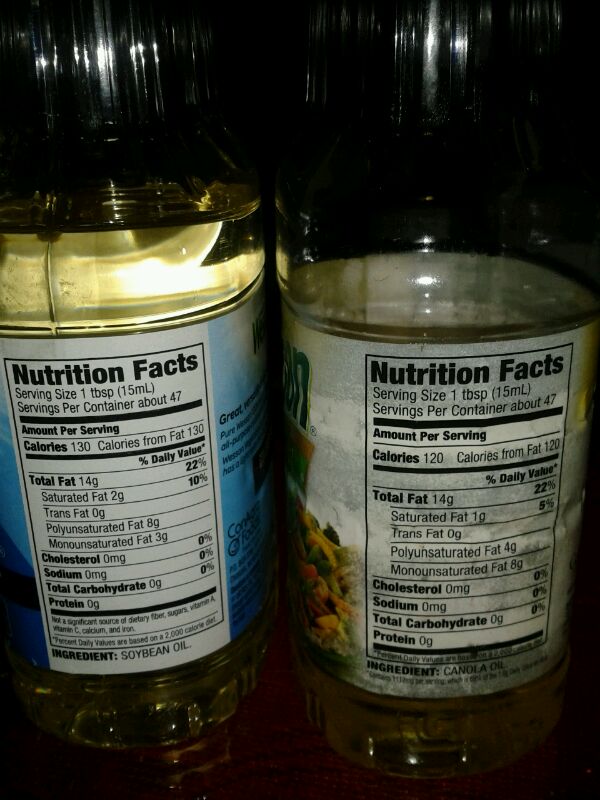In a dimly lit room, this photograph captures two bottles of vegetable oil standing side by side on a dark wooden shelf. The bottle on the left, almost full, displays a pristine blue label detailing its contents as soybean oil. The side panel includes the nutrition facts, noting each serving, a tablespoon, contains 130 calories from fat. In contrast, the bottle on the right is nearly empty, with a label visibly smeared with oil, giving it a gleaming appearance. This bottle is identified as canola oil, with its nutrition facts indicating a similar serving size yielding 120 calories from fat. Both bottles’ transparent plastic allows a clear view of their contents, encapsulated in the sparse lighting and dark ambiance of the setting.